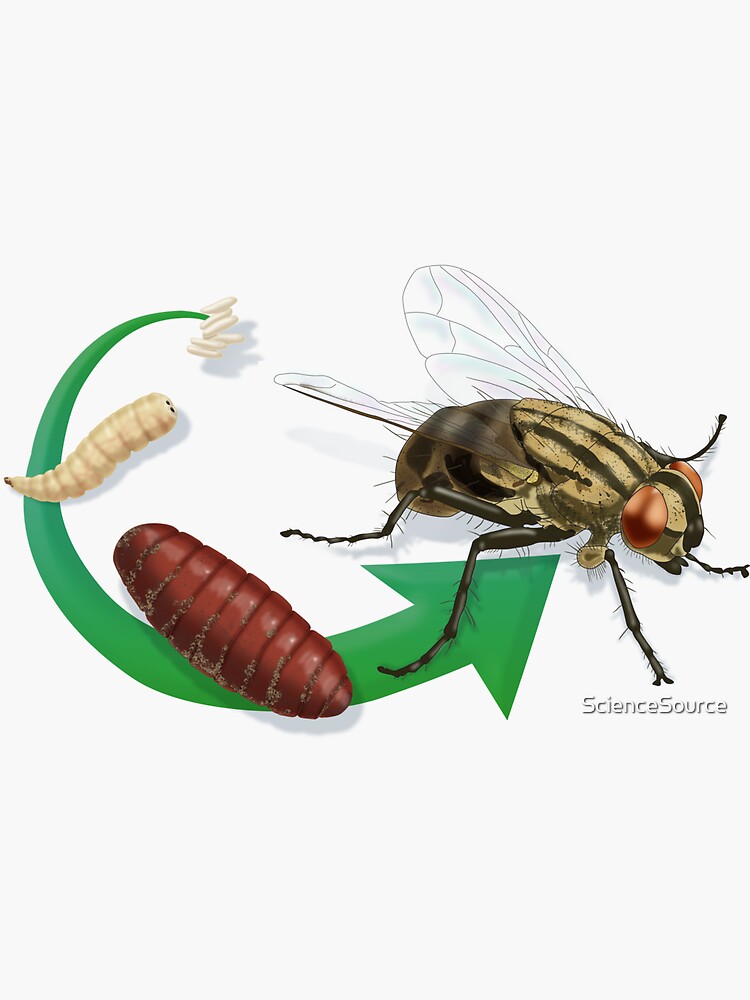This detailed illustration by Science Source depicts the life cycle of a fly, highlighting each developmental stage in a circular pattern emphasized by a green arrow. Starting from the left side, we first see small white eggs resembling rice grains. As the arrow curves and progresses, it points to a segmented yellowish larva, followed by a larger reddish-brown cocoon or chrysalis. The final stage, highlighted on the right side, showcases an adult fly in exquisite detail. The fly sports clear wings and has five visible hairy legs. Its body features tan and dark greenish-brown stripes, with the bottom portion being particularly dark green. The fly's most striking features are its huge copper-colored eyes and spiny tentacles, and it faces to the right as if ready to take off. The words "science source" are displayed underneath the fly in white text.